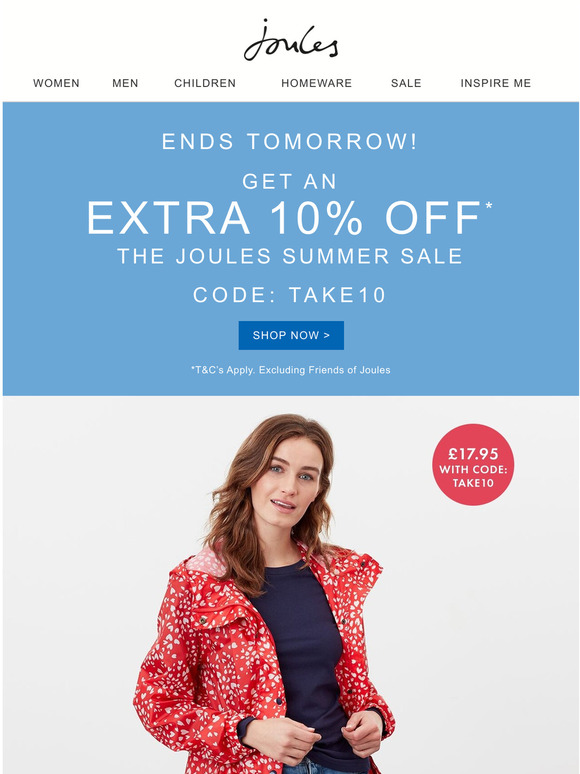The image is a detailed promotional banner for a website, displayed within a rectangular layout. At the top, the word "joules" is written in elegant black cursive lettering with a lowercase "j-o-u-l-e-s." Directly beneath this, there are subcategories in bold uppercase black letters: "WOMEN," "MEN," "CHILDREN," "HOMEWARE," "SALE," and "INSPIRE ME."

Below the navigation, a light blue rectangular background features the all-caps, white text: "ENDS TOMORROW!" followed by "GET AN EXTRA 10% OFF*" in prominent uppercase lettering. The phrase "THE JOULES SUMMER SALE" is displayed in bold letters beneath this. Below that, "CODE: TAKE10" is clearly indicated.

A blue rectangular button at the center reads "SHOP NOW >" in light blue. Underneath, in fine print, "T&C'S APPLY. EXCLUDING FRIENDS OF JOULES" is written, emphasizing terms and conditions.

At the bottom of the banner, a picture of a smiling Caucasian blonde woman is shown. She is wearing a navy blue shirt and holding a red jacket detailed with white polka dots. She also appears to be wearing jeans. In the top right corner of the photo, the price "£17.95" is displayed in white, followed by the promotional text "CODE: TAKE10" in white letters inside a red circle.